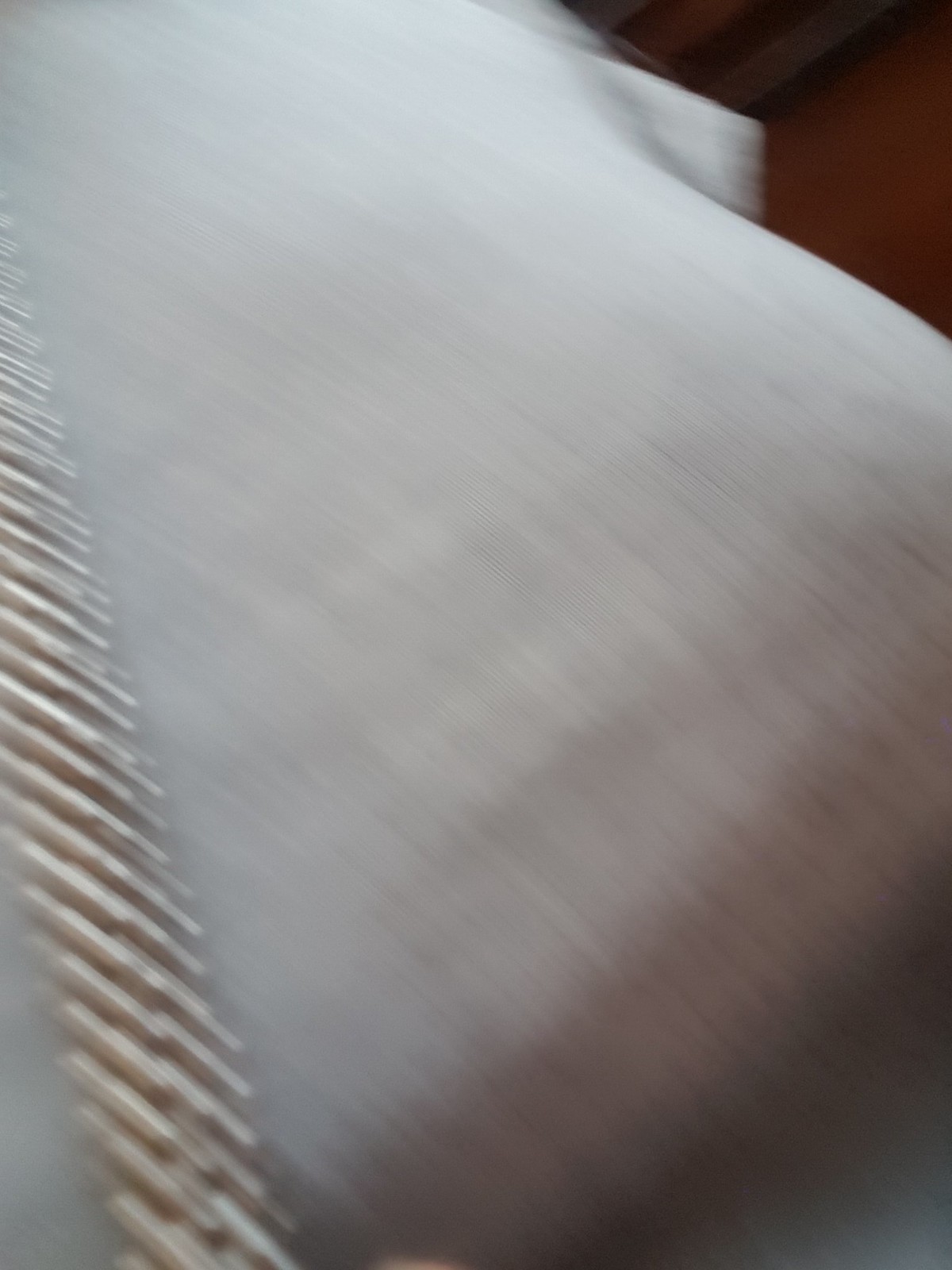This is a very blurry photo, likely taken inside a house, featuring a large, soft, and fluffy white object that appears to be a couch cushion or a corner of a bed with a white thin blanket draped over it. The main object, which resembles a rectangular cushion, occupies about 90% of the image. A gold or silver decorative rope-like piece is visible on top of the cushion. In the upper right-hand corner, a section of the brown wooden floor can be seen, along with a small part of what might be a brown wooden nightstand. The overall image is out of focus, possibly due to camera movement or low quality, making it challenging to discern finer details.